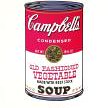This image showcases a detailed print or drawing of a classic Campbell's Condensed Old Fashioned Vegetable Soup can. The can is depicted with the brand's iconic red and white design, synonymous with Campbell's. The "Campbell's" name is elegantly written in cursive at the top, while "Condensed Old Fashioned Vegetable" is presented in clear, easy-to-read print. Although some additional text is present beneath the "Old Fashioned Vegetable" label, it is not legible in this representation. The illustration captures the typical silver aluminum hues at both the top and bottom edges of the can, highlighting its authentic appearance. This artwork celebrates the recognizable and timeless Campbell's soup can design.